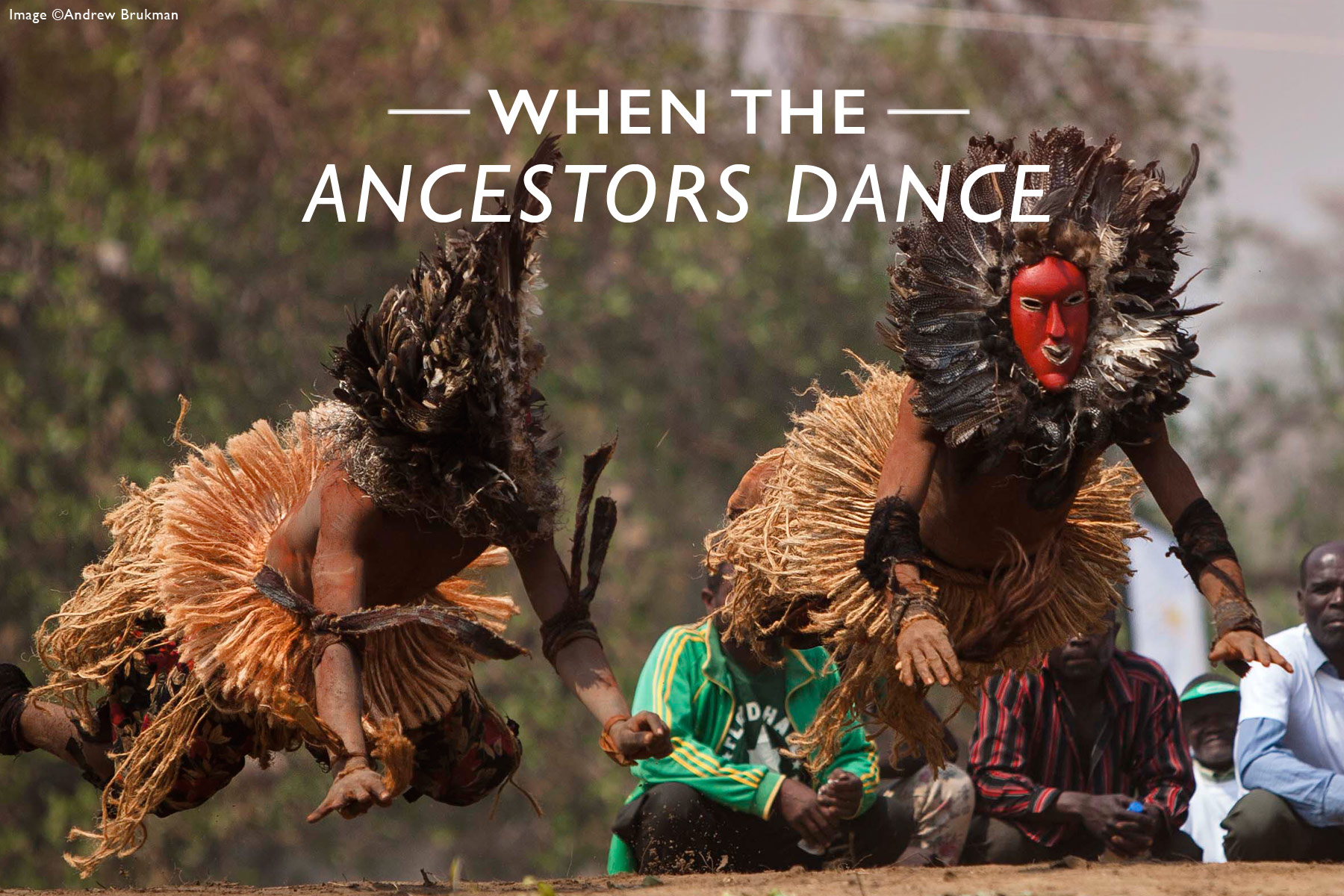The image depicts a vibrant ceremonial dance by a Native Indigenous tribe set outdoors amidst a backdrop of faded foliage and a grey building to the right. Central to the scene are dancers adorned with traditional costumes and face paint; one dancer's face is painted red, while another's is in black. Each dancer wears intricate masks framed by materials resembling a lion's mane, featuring dark brown and lighter colors, and they don fringed skirts in light tangerine hues composed of multiple strings. Their bare arms are decorated with braided ropes. The dancers perform dynamically on the ground, encapsulating the phrase "when the ancestors dance," which is prominently displayed in white letters. Observing this powerful moment are several individuals sitting on the ground, including three men in contemporary clothing—one in a black and red striped shirt, another in a lime green and yellow jacket, and a third in a long-sleeved shirt—captivated by the ancestral performance.